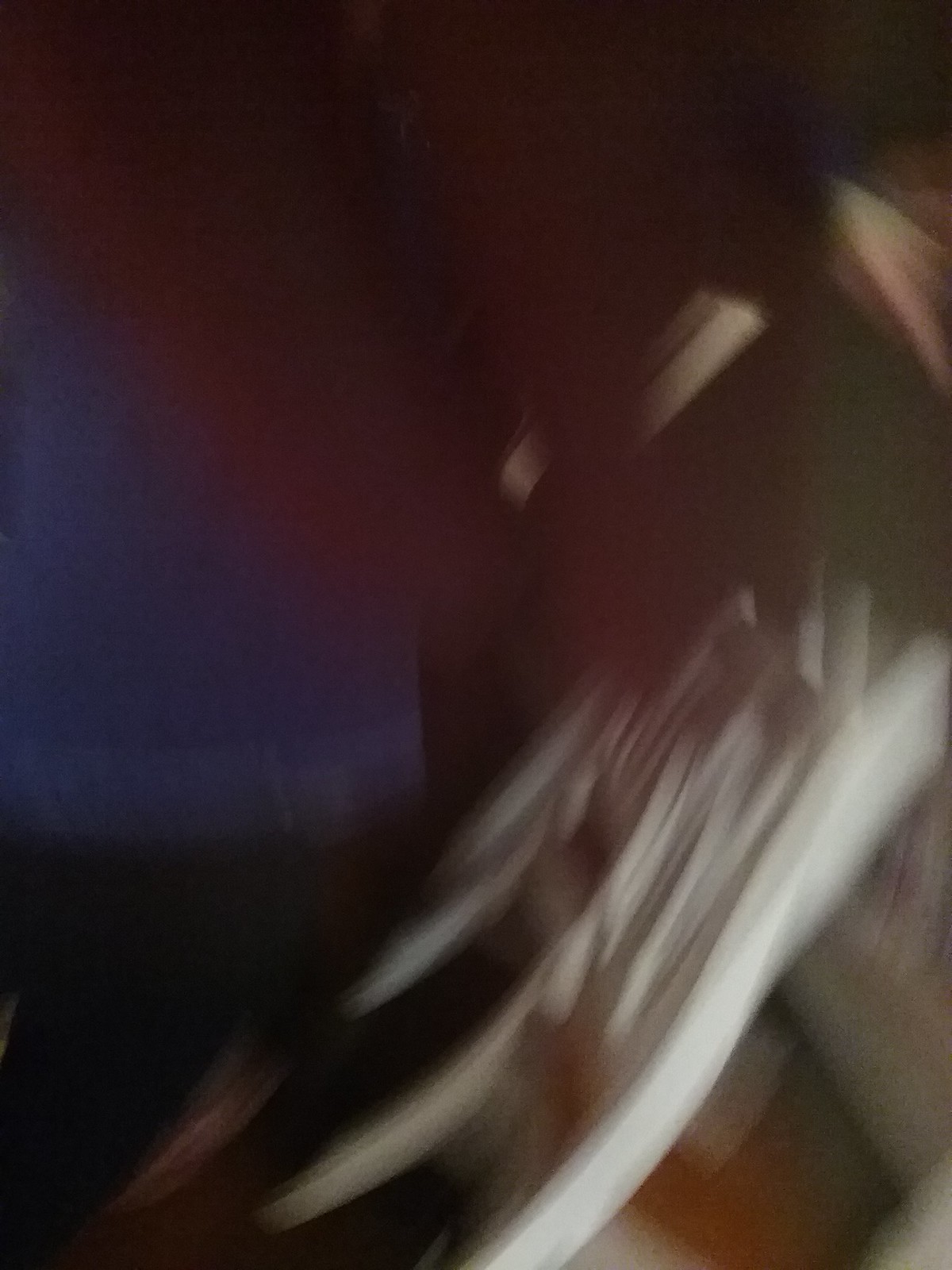This is an extremely blurry color photograph rendered almost entirely unintelligible due to the lack of clarity. The composition features a prominent dark blue area on the far left side, while a whitish element extends down from the right toward the bottom center of the image. At the top, there's a reddish swirl which might be someone's fingers partially obstructing the lens, though the overall haze makes this difficult to confirm. The photograph is predominantly dark-hued and exhibits a taller-than-wide aspect ratio. There is no text or recognizable object within the frame, leaving the subject matter ambiguous and unclear.